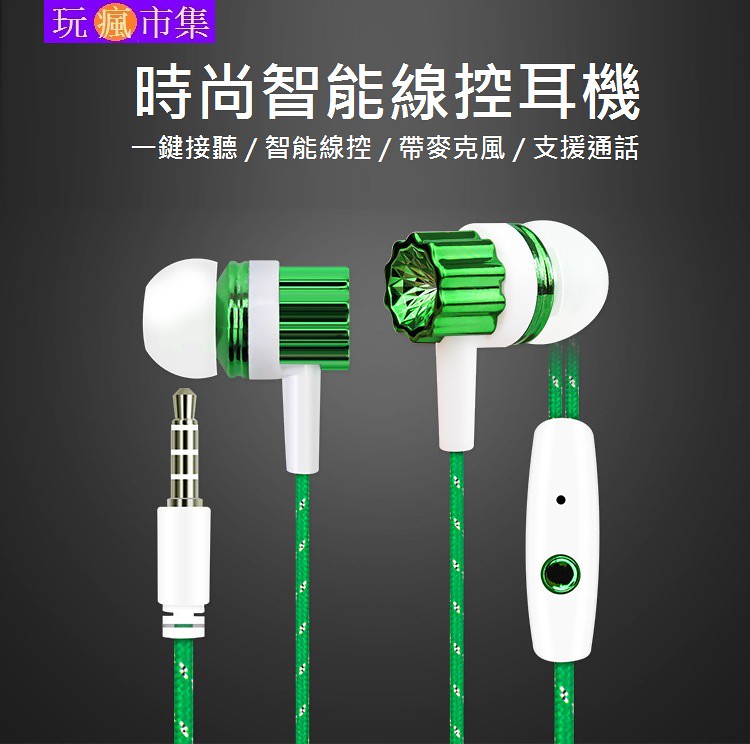This is a detailed advertisement image for wired earbuds set against a black background that transitions to dark gray in the center. At the top left corner of the image, there is a purple box with light pink lettering, featuring an orange sun-like logo with additional unreadable characters. The main highlight of the advertisement is large white text printed prominently across the gradient background. The focal point of the image is a close-up of the white earbuds adorned with shiny high-polished, gem-like green details. The earbuds are connected via bright green, fabric-covered cables. One cable features an integrated microphone while the other ends in an RCA plug for connectivity. Various features of the earbuds are described in a foreign, possibly Asian script, showcased throughout the image.